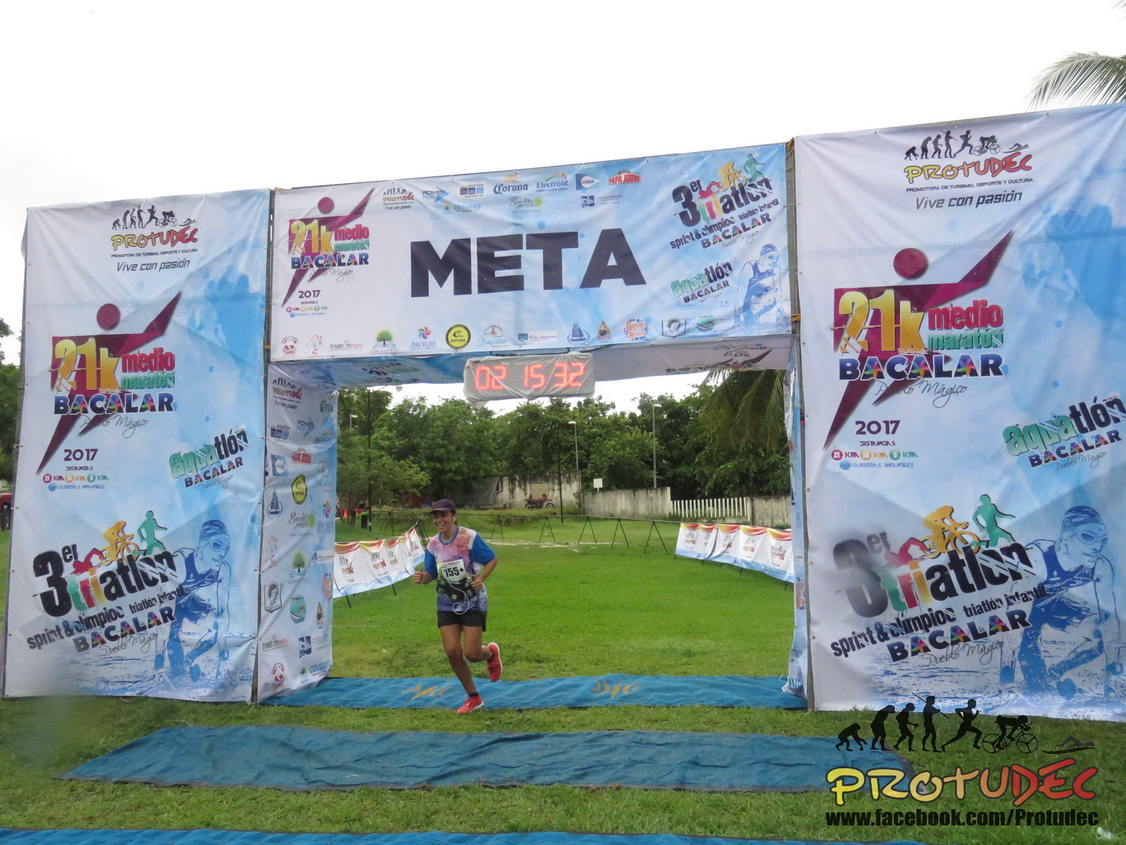The image captures a woman crossing the finish line at a triathlon race. The finish line banner prominently displays the word "META" in black on a white and blue background. The timer above the archway reads 2 hours, 15 minutes, and 32 seconds. The woman, wearing a blue printed top, short black shorts, red-orange sneakers, and a black hat, appears to be in motion with headphones on. She bears the number 155 on her shirt. In the lower right corner of the image, there is a logo for Pro2Deck, accompanied by images depicting people transitioning between swimming, cycling, and running. The scene is set in an outdoor area with grass, a fence, and a tree line in the background. The ground shows two red and two blue mats for the participants to cross. Various colorful banners and logos, including ones for Bacalar and Pro2Deck, are visible around the space, adding vibrancy to the energetic atmosphere of the event.